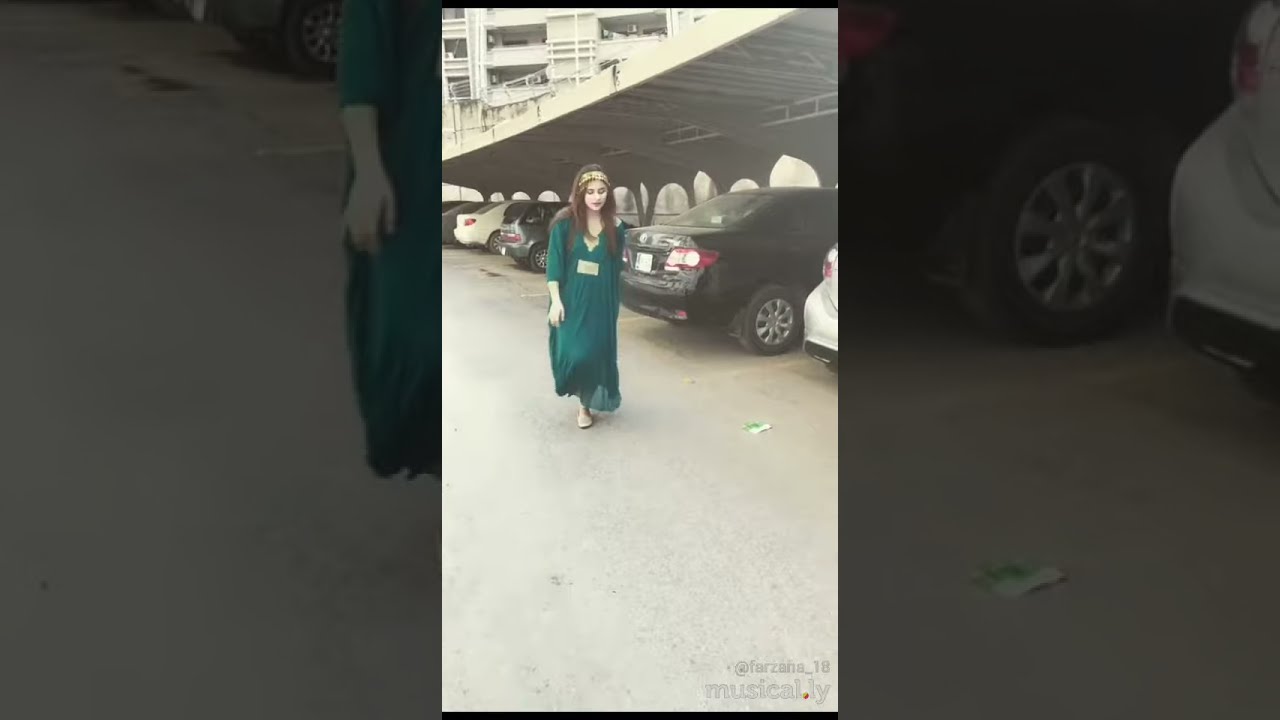In this vertically oriented, overexposed photograph with a unique blend of black-and-white and faded color, the central focus is a young woman walking towards the viewer in an outdoor parking lot. She is adorned in a long, flowing, traditional Middle Eastern green dress that reaches her ankles and a gold headband that complements her long brown hair cascading past her shoulders. Her gaze is directed downward, adding a subtle depth to her expression.

The background features a row of parked cars on the right, sheltered by a concrete overhang with arches lining the wall behind them. In the distance, apartment buildings are faintly visible amidst the muted colors. The photo itself appears as the central piece within a collage, bordered by enlarged sections of the same image on either side—on the left, the woman’s arm and dress are visible, while on the right, parts of the cars are seen.

There is minimal color in the image except for the woman's green dress and faint red in a car taillight. Below the photograph, in the bottom corners, are a partially obscured username, “@farzana_18,” and the logo “musical.ly,” serving as subtle identifiers.